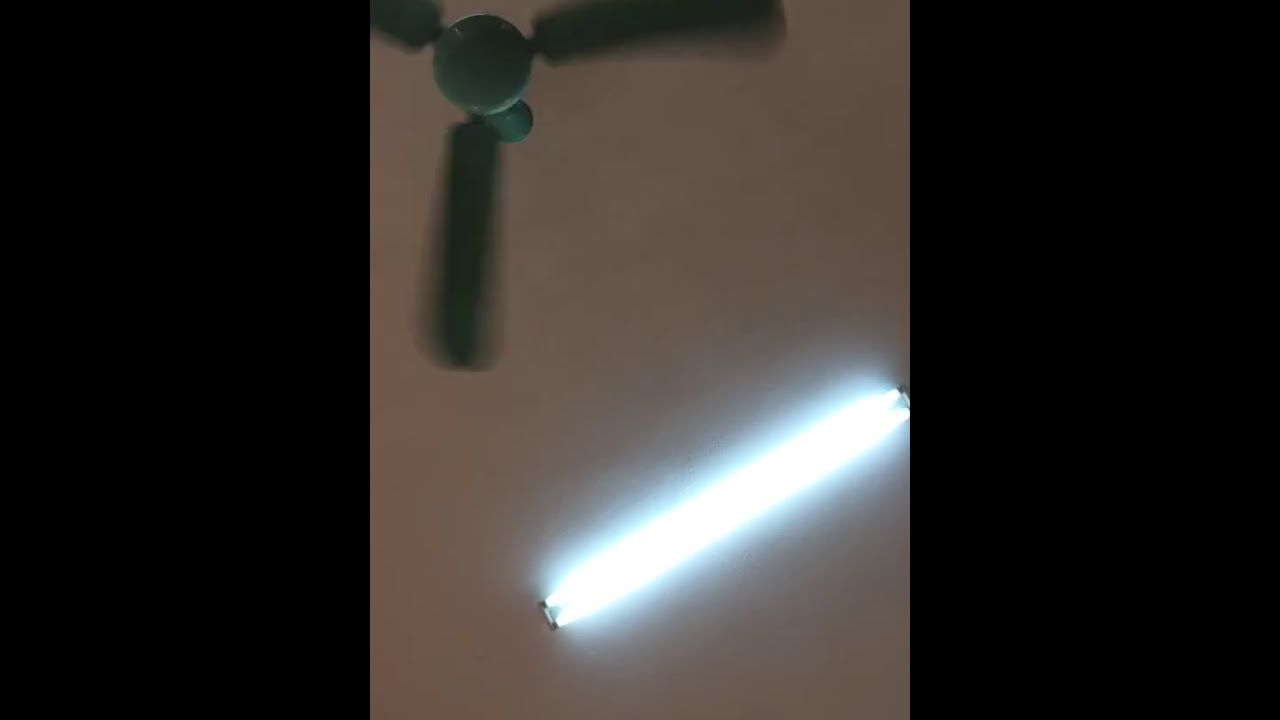This detailed and textured image captures the scene of an indoor ceiling, likely in someone's home, viewed from a low angle pointing upward. The focus is on a beige or off-white ceiling that features a dark, three-pronged ceiling fan in motion in the upper left corner. The fan has black and gray blades, appearing slightly blurred due to its rotation. In the lower right corner, there is an illuminated, double-tubed fluorescent light fixture, distinguished by its bright white center and a softly diffused neon blue glow around its edges. The photograph is bordered by thick black strips on both the left and right sides, drawing attention to the central portion of the image. The overall setting is a residential indoor space, with prominent color themes of beige, white, black, and metallic hues such as silver or copper.